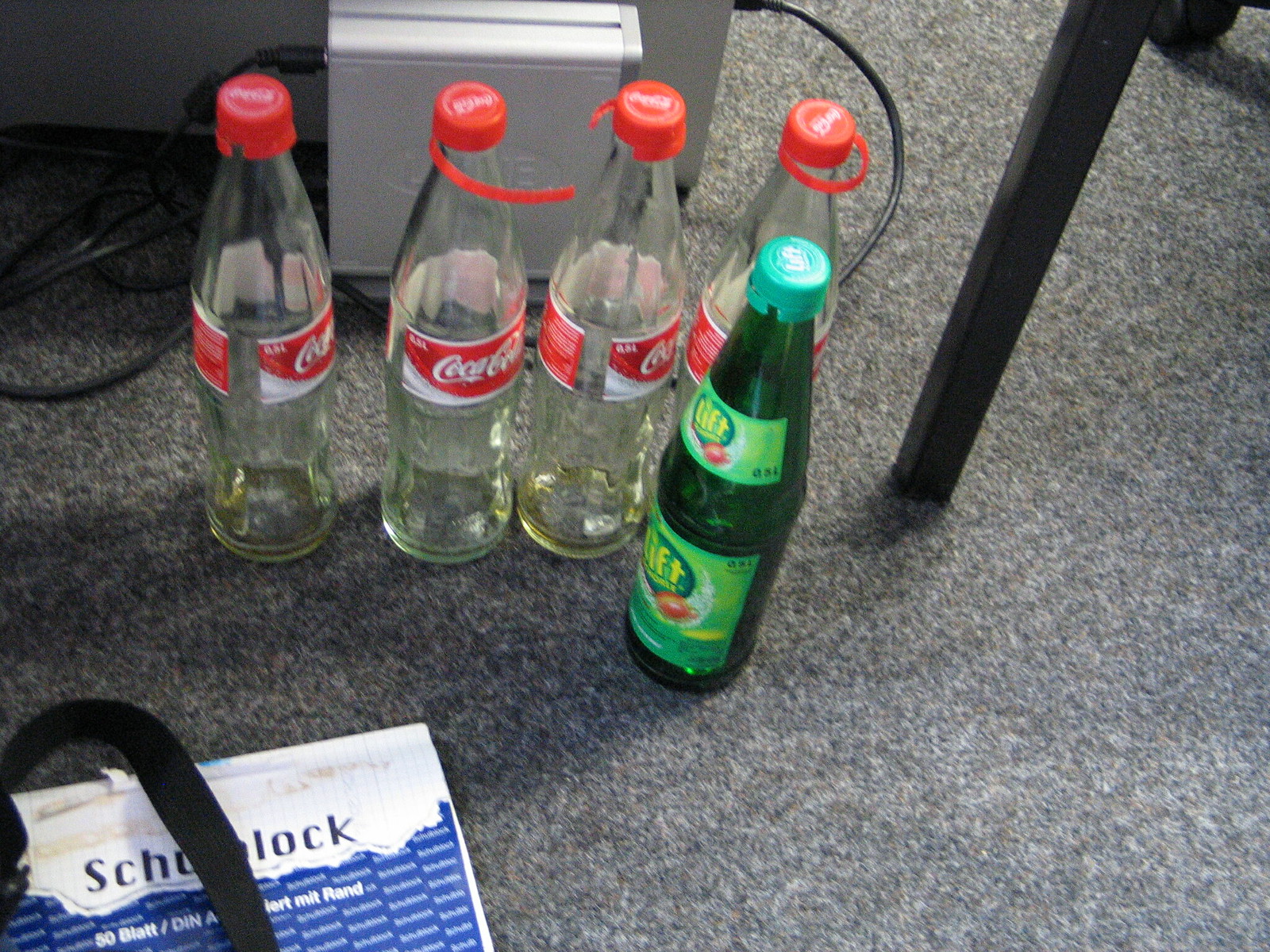This photograph captures a cluttered section of an office with a short napped, gray carpet featuring a light brown and white pattern. Dominating the center are five bottles arranged on the floor. Four of these are empty, classic glass Coca-Cola bottles with red and white labels and red plastic caps, some of which are twisted off and stretched out. Among them is a distinctive green glass bottle with a green cap and a label reading "Lift" in yellow letters; this bottle appears to contain some remaining liquid. To the left sits a blue and white reusable shopping bag partially covered by a black strap or rope, while a nest of black cables lies in the top left corner. Also visible is a grey computer router positioned near the bottles, and a lone black chair leg extends into the frame from the top right.